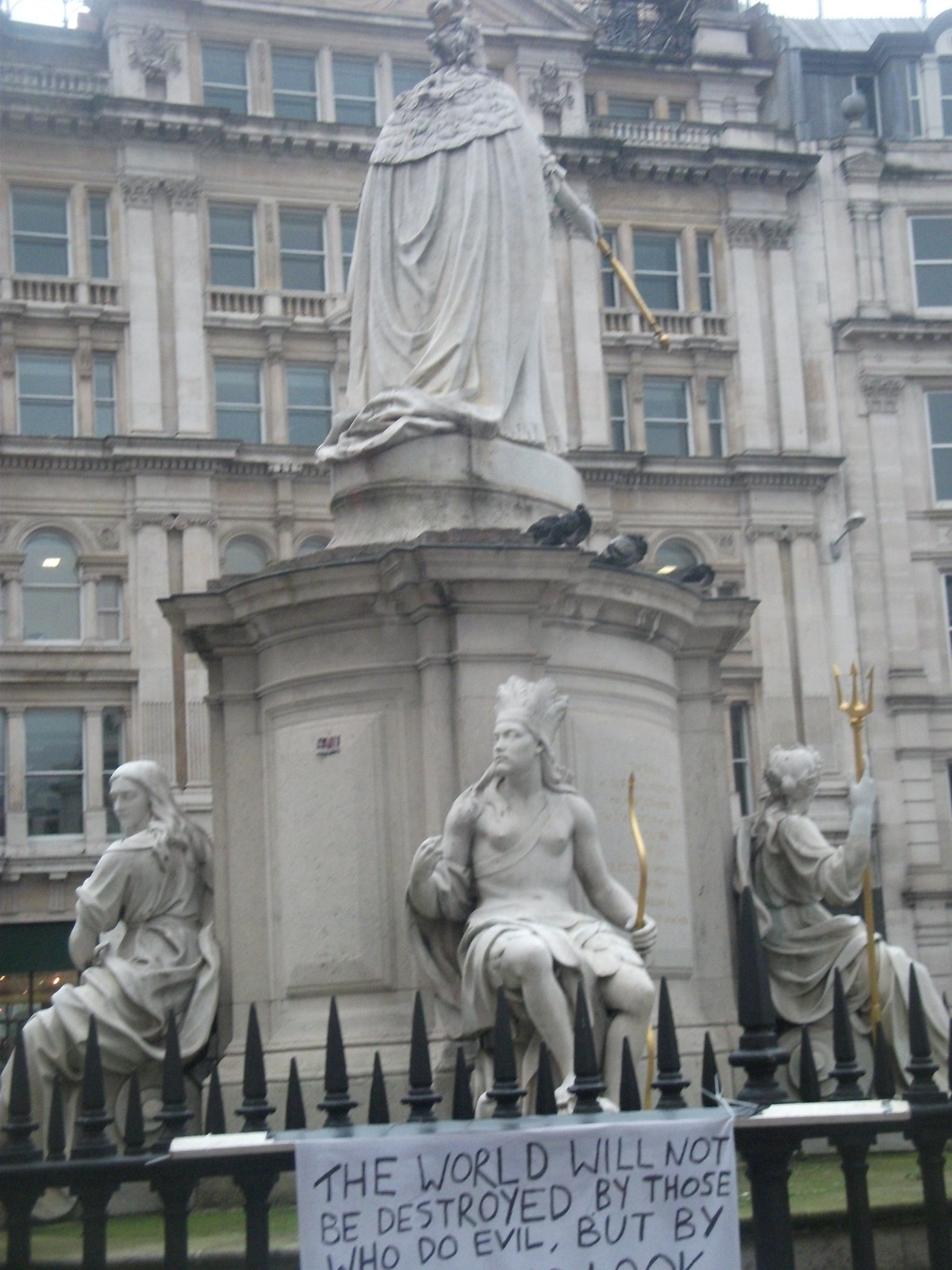This photograph captures a large, intricately detailed statue set in a European urban courtyard, likely in front of a substantial stone building resembling an apartment or government building. The primary figure atop the statue is a monarch, either a king or Queen Anne, distinguished by a crown and a flowing cape, holding a golden scepter or sword extended forward. The monarch stands on a round pedestal elevated above a larger, darker stone base.

Surrounding the larger pedestal are three seated statues, each depicted as royal guards. The guard on the left, partially obscured, appears to hold a golden weapon, possibly a trident or pitchfork. The central guard is more visible, wielding a golden bow and adorned with a crown, while the guard on the right holds another golden weapon, potentially a spear. These statues are arranged facing different directions, possibly symbolizing vigilance from all sides.

In front of the statue stands a black wrought iron fence with pointed spikes, and affixed to it is a white paper sign with a handwritten message in black marker. The sign reads: "The world will not be destroyed by those who do evil but by," with the remainder of the message cut off. 

Above the guards, near where birds are perched, the monarch remains the focal point, indicating their supreme authority. The background reveals a tall, stone building with multiple stories, likely five or six, featuring tall, vertical rectangular windows separated by Doric columns, contributing to the grand, historic ambiance of the scene.